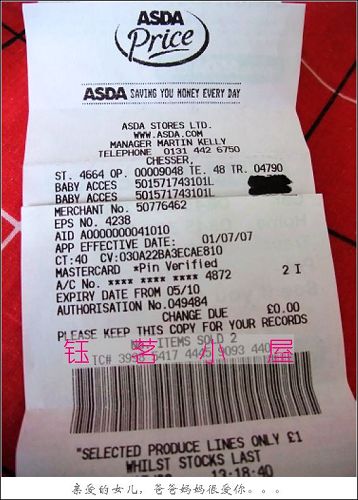On a predominantly red background with interspersed black and white lines, there is a prominently displayed white receipt. The top of the receipt features bold black text stating "ADA, ASDA Price." Below this, it reads "ASDA, Saving you money every day." Further down, the receipt indicates "ASDA Stores LTD" with their website, www.asda.com. The managerial contact is listed as "Manager: Martin Kelly," followed by the telephone number "0131-442-6750."

The receipt includes specific transaction details such as "Baby Access," "Merchant Number APS Number: 42328ID," "App Effective Date: 01-07-07," and "CT.40CV." It also mentions "Mastercard," an "Authorization Number," and an "Expiry Date: 05-10." At the bottom of the receipt, it advises to "Please keep this receipt for your records."

There are some Asian characters printed, and above the barcode, there is pink text that reads "Selected Produce Lines Only."